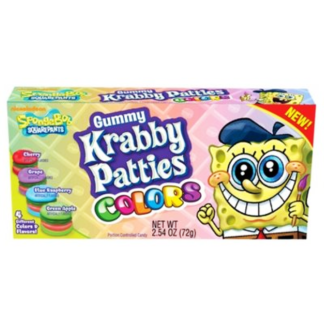The image showcases a box of Gummy Krabby Patties, a colorful candy product prominently featuring the SpongeBob SquarePants theme. The packaging is vibrant and eye-catching, adorned with a playful mix of yellow, pink, and pastel hues. The brand name "Gummy Krabby Patties" is displayed in playful white text set against a purple background, while the word "colors" is creatively spelled out with each letter in a different shade: green, red, orange, blue, yellow, and purple. The top left corner of the box bears the Nickelodeon logo and the SpongeBob SquarePants title, promoting the beloved children’s show.

On the far right side of the packaging, SpongeBob himself is depicted with a big, cheerful smile, blue eyes, and holding a paintbrush, donned in a blue artist's beret. The top right corner features a "new" label in a red triangle with yellow text. The image also includes visuals of the Gummy Krabby Patties in various flavors: cherry (red bun), grape (purple bun), blue raspberry (blue bun), and green apple (green bun). This delightfully colorful and engaging packaging is clearly designed to attract children and fans of SpongeBob SquarePants, making it a tempting treat for young ones and nostalgic adults alike.